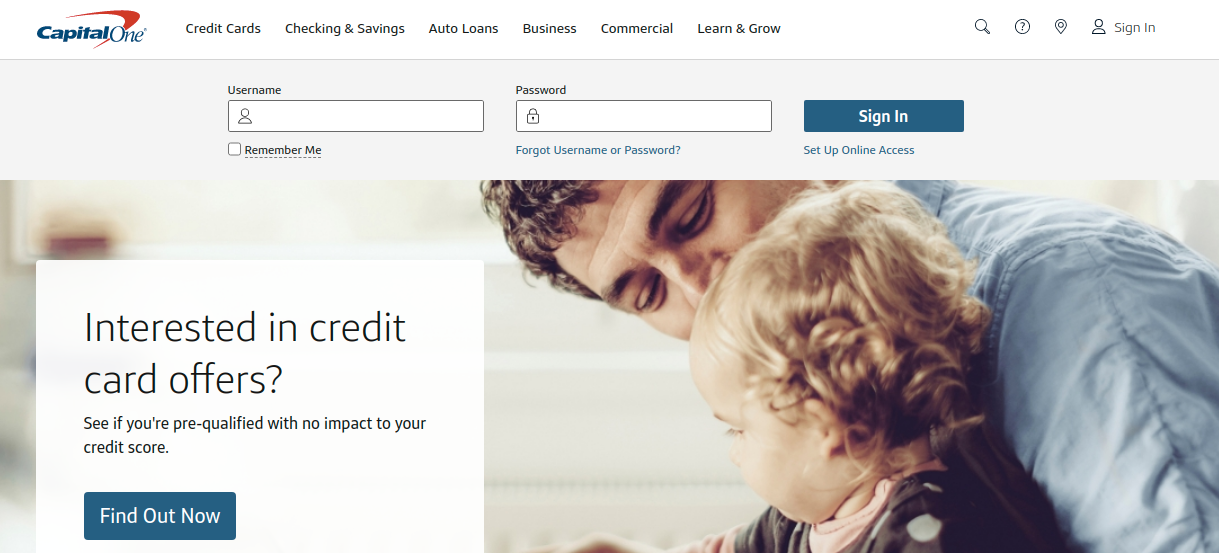The homepage of the Capital One website prominently features a large, heartwarming image of a father lovingly kissing his son on the temple as the child plays. Positioned at the upper left corner is the recognizable Capital One logo, accompanied by a menu bar offering navigation options for various services such as Credit Cards, Checking & Savings, Auto Loans, Business, Commercial, and Learn & Grow. 

Additional navigation features are present, including options to search, ask questions, locate a nearby branch, and sign in. The focus of the page is the sign-in section, where users can enter their username in a designated box followed by an option to select "Remember Me" for future visits. Below it, the password box is situated, along with hyperlinks for forgot username or password recovery. A prominent blue 'Sign In' button awaits to be clicked once credentials are entered, and there is an additional hyperlink below labeled 'Set up online access' for new users to get started.

A discreet white box overlays part of the main image, inviting visitors to explore credit card offers with a prompt reading, "Interested in credit card offers? See if you're pre-qualified with no impact to your credit score." This section includes a blue 'Find Out Now' button for users to click and learn more.